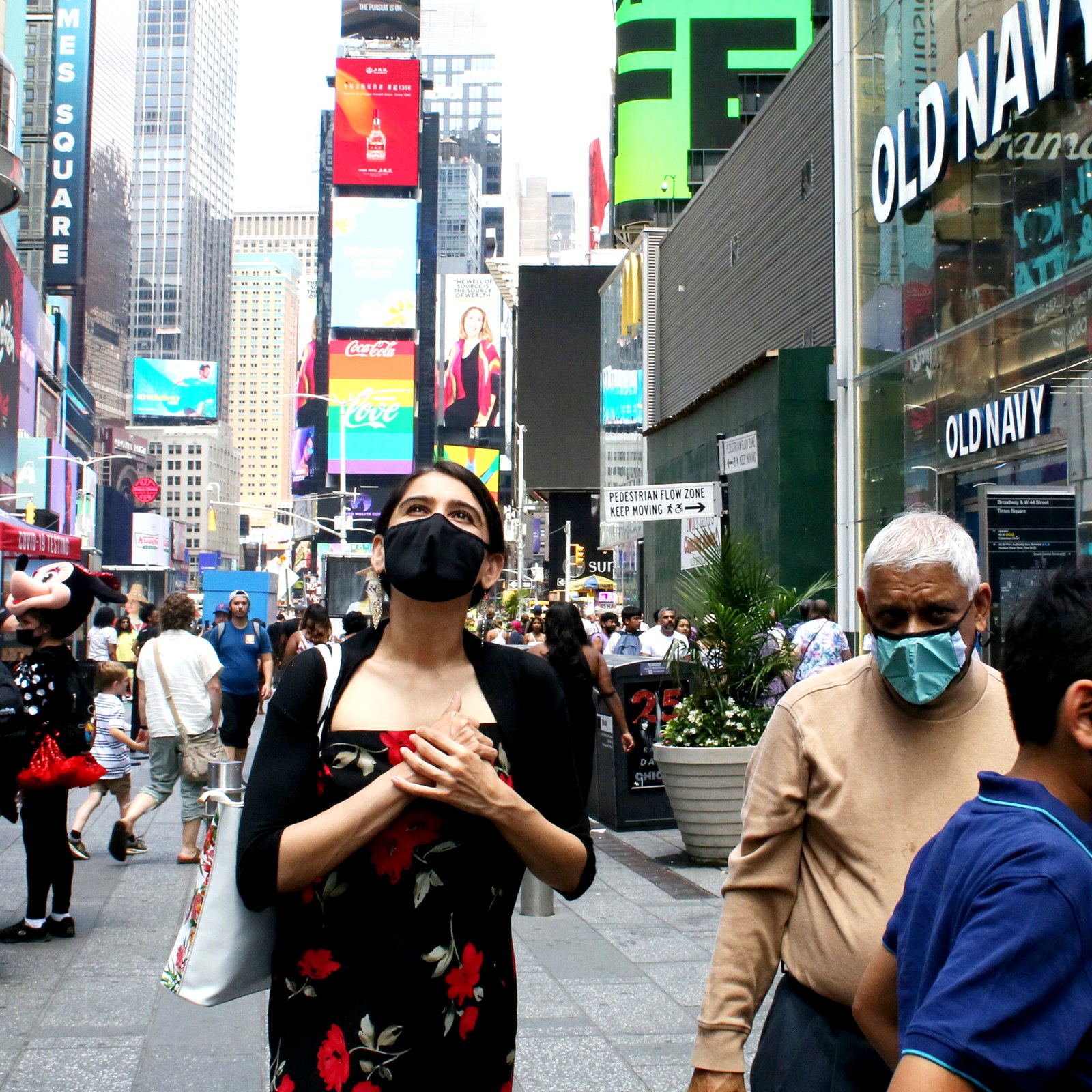In the heart of Times Square, New York City, a woman walks with an air of quiet determination. She is dressed in a striking red dress adorned with a delicate floral pattern that contrasts vividly against the bustling urban backdrop. Clad in a black face mask emblazoned with the words "Old Navy, New Orleans," she clasps her hands gently at her front. Her eyes, partially visible above the mask, seem to radiate a sense of hope and optimism as she navigates through the iconic, neon-lit landscape. The scene captures a poignant moment of personal resilience amidst the ceaseless energy of the city.